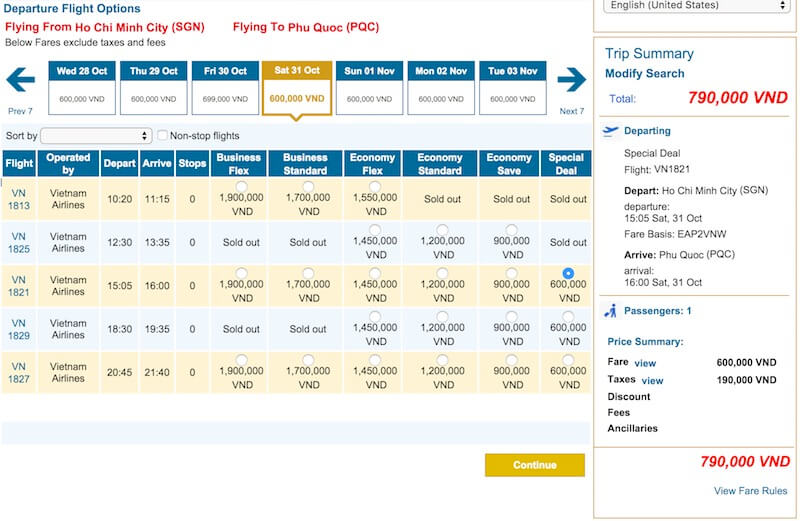On a white background, at the upper left corner in blue text, it reads "Departure Flight Options." Below this, in black text, it states "Flying from Ho Chi Minh City" and "Flying to Phu Quoc, Phu Quoc." A note beneath mentions, "Below fares exclude taxes and fees." 

Next, a blue arrow points to the left with the text "Previous 7" underneath it. Below this, a list of dates follows: "Wednesday, October 28th, Thursday, October 29th, Friday, October 30th, Saturday, October 31st, Sunday, November 1st, Monday, November 2nd, and Tuesday, November 3rd." Each date shows a price of 600,000 VND (Vietnamese Dong).

There is an option to "Sort by" and all available flights are listed under Vietnam Airlines. The flight times range from 10:20 AM to 8:45 PM. 

One flight has been selected, with a total cost of 790,000 VND. This amount includes the fare, taxes, and fees for a special flight route from Ho Chi Minh City to Phu Quoc. The selected fare and total price of 790,000 VND are reiterated at the bottom of the image.